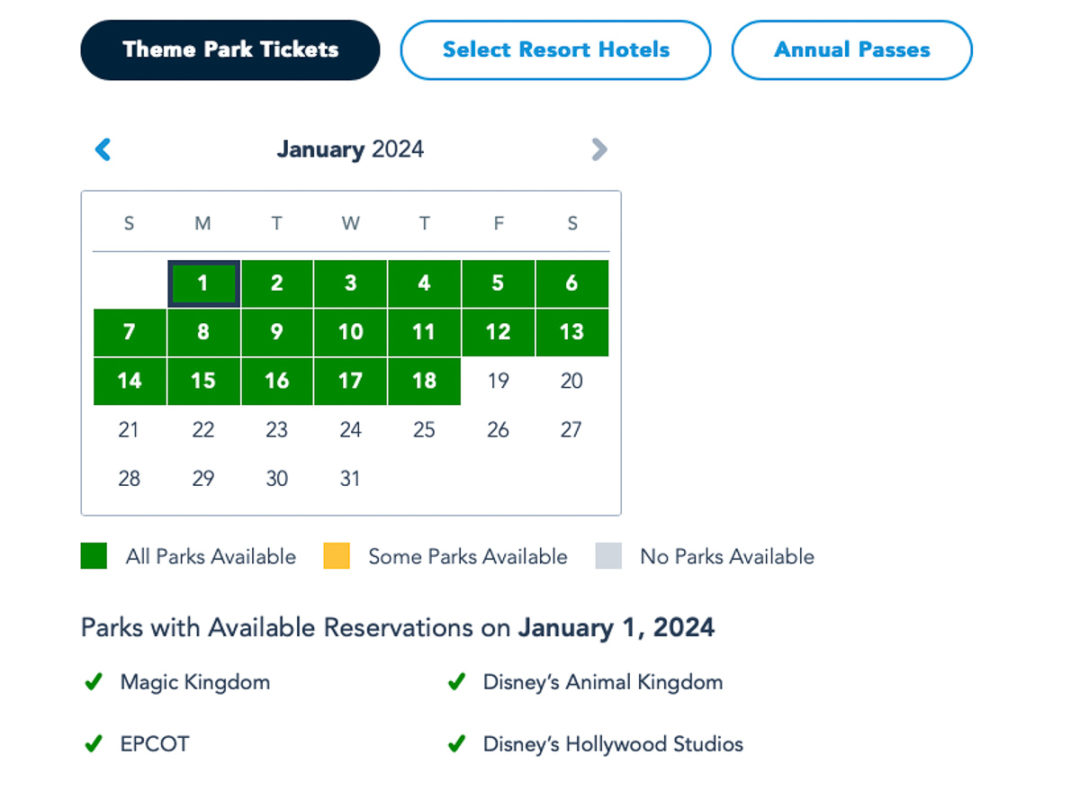The image depicts a section of the Disney website where users can purchase theme park tickets, specifically for visitors staying at select resort hotels or those holding annual passes. The main feature of the image is a calendar for January 2024, allowing users to select their desired visitation dates. The calendar displays the dates from Sunday, January 1st, through Wednesday, January 31st, with availability marked in different colors: green for all parks available, yellow for some parks available, and gray for no parks available. The overall design uses white text on the calendar. Beneath the calendar, there is a legenda clarifying the color codes, and a specific note for January 1st, 2024, indicating that all four main Disney parks—Magic Kingdom, Disney's Animal Kingdom, Epcot, and Disney's Hollywood Studios—have available reservations.